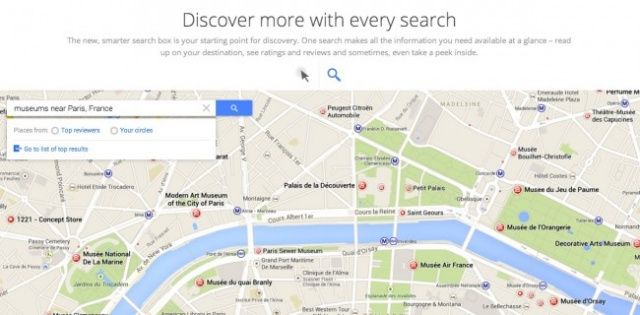Screenshot of a map showing a search for museums near Paris, France. The search menu, positioned above the map, features options for top reviewers in the user’s circle and includes a blue button labeled "Go to the top results." At the top of the screen, a tagline reads: "Discover more with every search," promoting a new Smarter Search box designed to provide comprehensive information at a glance. Users can read about destinations, see ratings and reviews, and sometimes even take a virtual peek inside places. The search bar prominently displays the text, "museums near Paris, France," and an adjacent cursor. The map centers around an area in Paris close to the river, potentially near notable landmarks. Despite some text being difficult to read, the image suggests functionality for exploring and discovering museums in the vicinity of Paris, France.